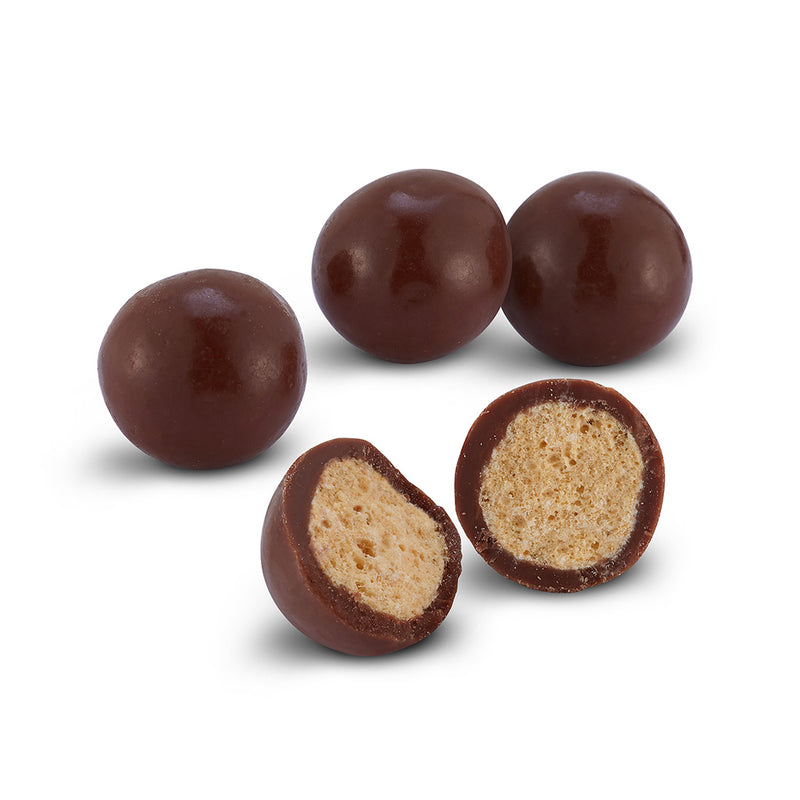The image features four milk chocolate-covered malted milk balls, arranged with three whole pieces in the back and one piece in the front that’s cut in half, yielding five visible items. The chocolates resemble Maltesers in size and shape but differ with a light brown, soft-looking interior rather than gooey. The cut chocolate reveals a slightly uneven cross-section displaying the crunchy malted center and crumbs around it. The chocolates have a shiny exterior that reflects light, giving a professional and polished presentation. The background is pure white, enhancing the chocolates' shadows and highlights, suggesting this is a product image likely produced by a manufacturer or retailer.